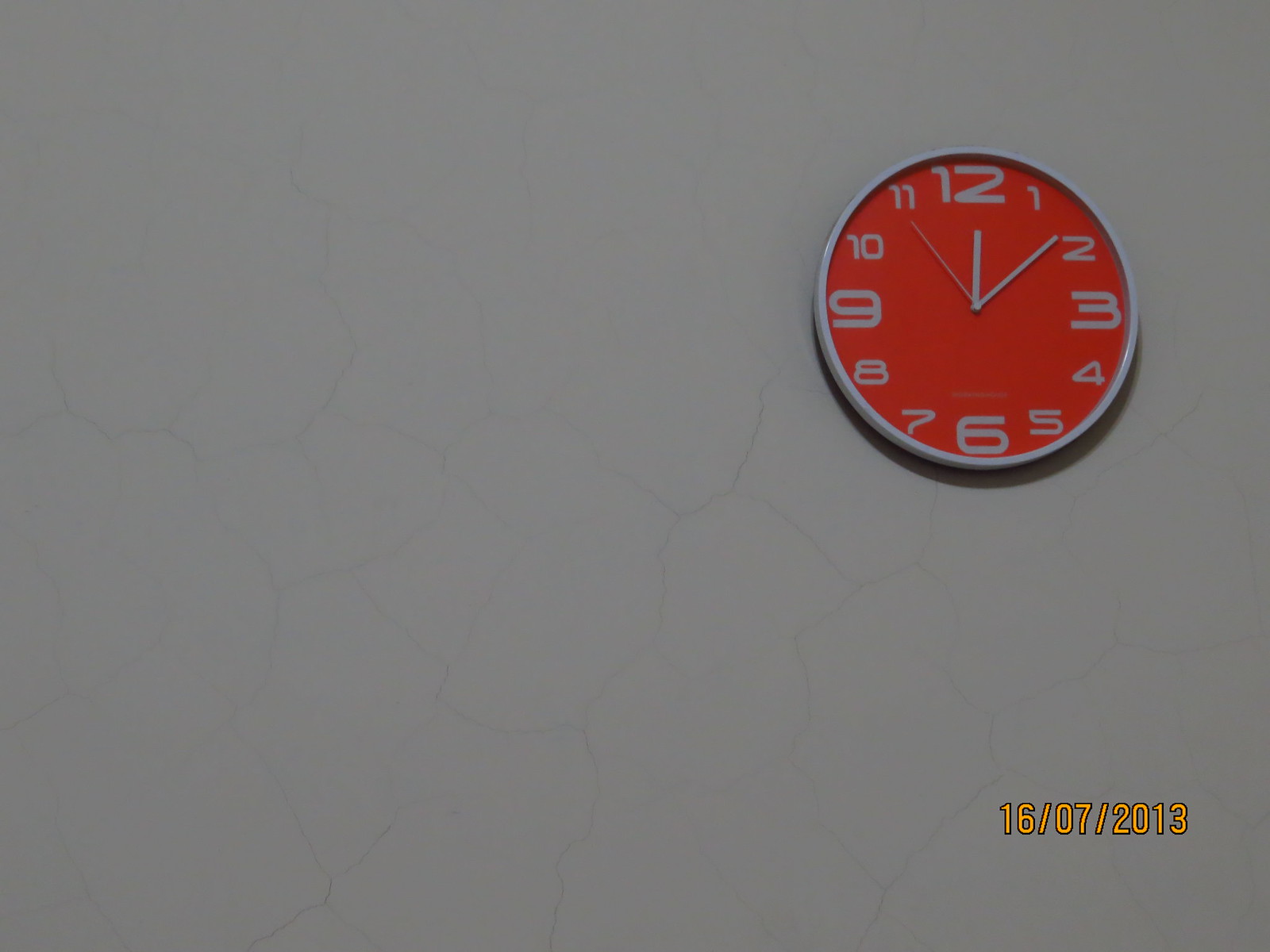This photograph captures a circular wall clock prominently displayed on a light grey wall featuring a subtle marbling pattern. The clock, which appears to have a silver or white metallic outer ring, contrasts sharply with its bright orange face. The hour and minute hands, along with the second hand, are all in a uniform white or grey color. The clock uniquely displays the numerals, with the 12, 3, 6, and 9 significantly larger than the other numbers. Additionally, a digital print at the bottom of the image reads "16-07-2013," indicating the date, which aligns with the time shown on the clock as 12:09. The setting appears to be indoors, and the overall simplicity of the photograph highlights the clock against the somewhat distressed, cracked wall.